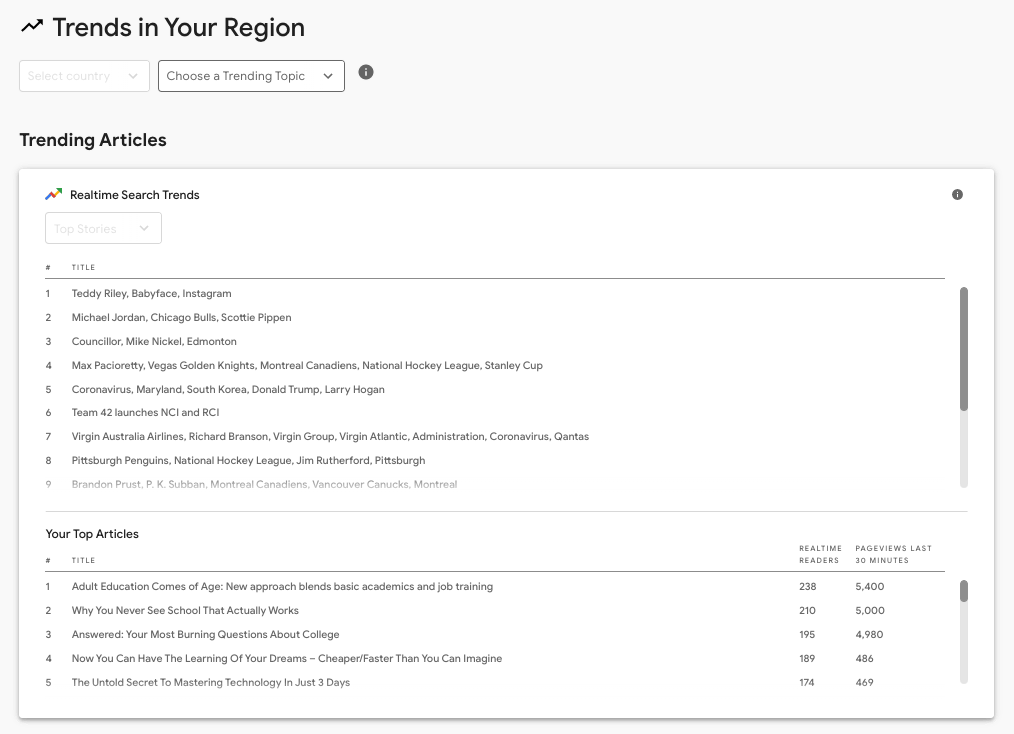Screenshot of the Google Trends webpage focusing on regional search analytics. 

In the top left corner, there is a section labeled "Trends in Your Region," accompanied by a black, squiggly arrow pointing to the right. Directly below this section are two drop-down boxes: the first is labeled "Select Country" but appears grayed out, and the second is labeled "Choose a Trending Topic."

Beneath these drop-down boxes, the section titled "Trending Articles" is prominently displayed in bold black font. Below this heading is a large white panel divided into two primary sections.

The top left of the panel displays "Real-Time Search Trends" with a drop-down box labeled "Top Stories," which is also grayed out. This panel contains two main sections, each featuring its own vertical scroll bar on the far right side.

The first section is titled "Title" and lists trending search topics such as:
1. Teddy Riley and Babyface Instagram
2. Michael Jordan, Chicago Bulls, and Scottie Pippen

The second section is titled "Your Top Articles," showcasing entries like:
- "Adult Education Comes of Age: New Approach Blends Basic Academics and Job Training."

This article notes real-time readership metrics, indicating the number one article has 238 real-time readers and accrued 5,400 previews in the last 30 minutes.

The overall layout is designed to provide a comprehensive overview of current and trending search topics, regional trends, and real-time article engagement.